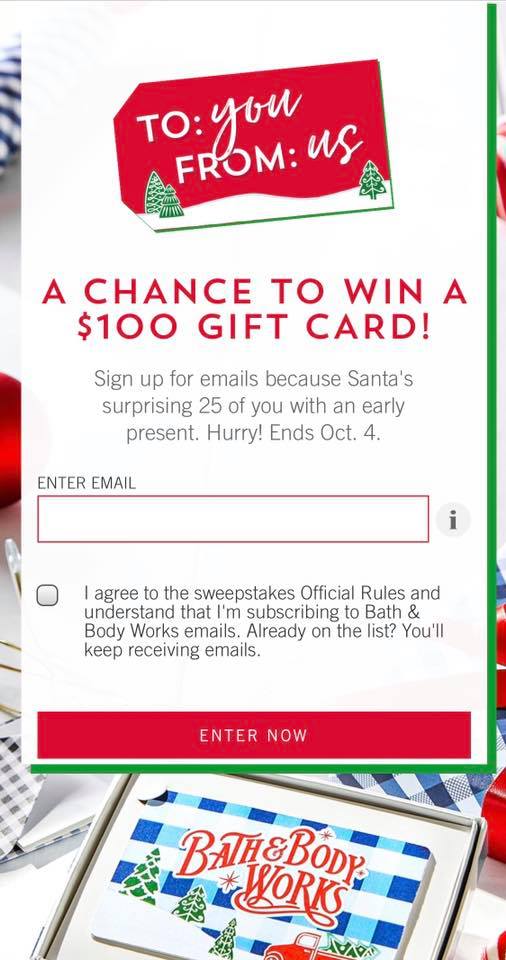The image features a festive background adorned with Bath & Body Works decorations. The backdrop showcases a dark and light blue and white plaid design, with the iconic "Bath & Body Works" logo in bold red letters. Adding to the holiday spirit, the scene includes decorative elements such as trees and a red truck, all set against a snowy ground.

Prominently displayed above this background is a white box, which has a green border along the bottom and right edges. The top of the box features a red banner with illustrations of three trees and some snow, and it bears the message "To You From Us." Below this, in bold red capital letters, the text announces, "A Chance to Win a $100 Gift Card." 

Further down, in gray text, it reads, "Sign up for emails because Santa is surprising 25 of you with an early present. Hurry, ends October 4th." Beneath this, there is a text box labeled "Enter Email," accompanied by a gray circle with a lowercase 'i' in the center, likely indicating additional information.

Below the email entry section, there is a checkbox next to the statement, "I agree to the sweepstakes official rules and understand that I'm subscribing to Bath & Body Works emails." Additional text reassures that if you are already on the list, you will continue receiving emails. Toward the bottom of the box, a bright red button prompts, "Enter Now."